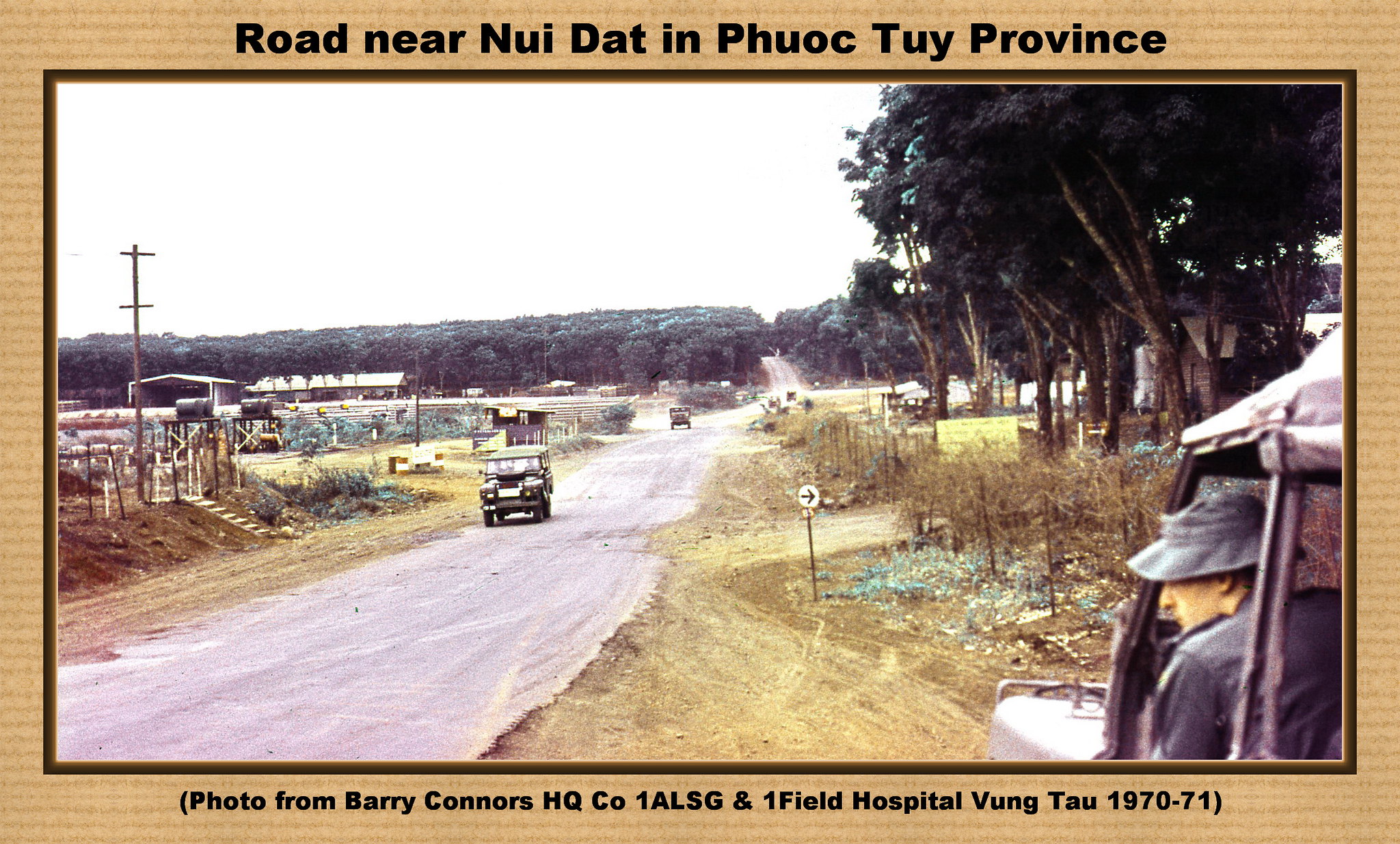This horizontal rectangular photograph, bordered by a beige frame, depicts a dirt road set in Vietnam, near Nui Dat in Phuoc Tuy Province, during the years 1970-1971. The road, flanked by dirt trails, stretches into the distance with an abundance of trees under a white sky. Two green Jeep-like vehicles are visible; one is driving down the unpaved road while the other, parked on the right, has a person wearing a bucket hat in the driver's seat. The photograph is credited to Barry Connors, HQ, 1 ALSG, and Onefield Hospital, Vung Tau, as indicated by the black writing on the top and bottom of the frame.